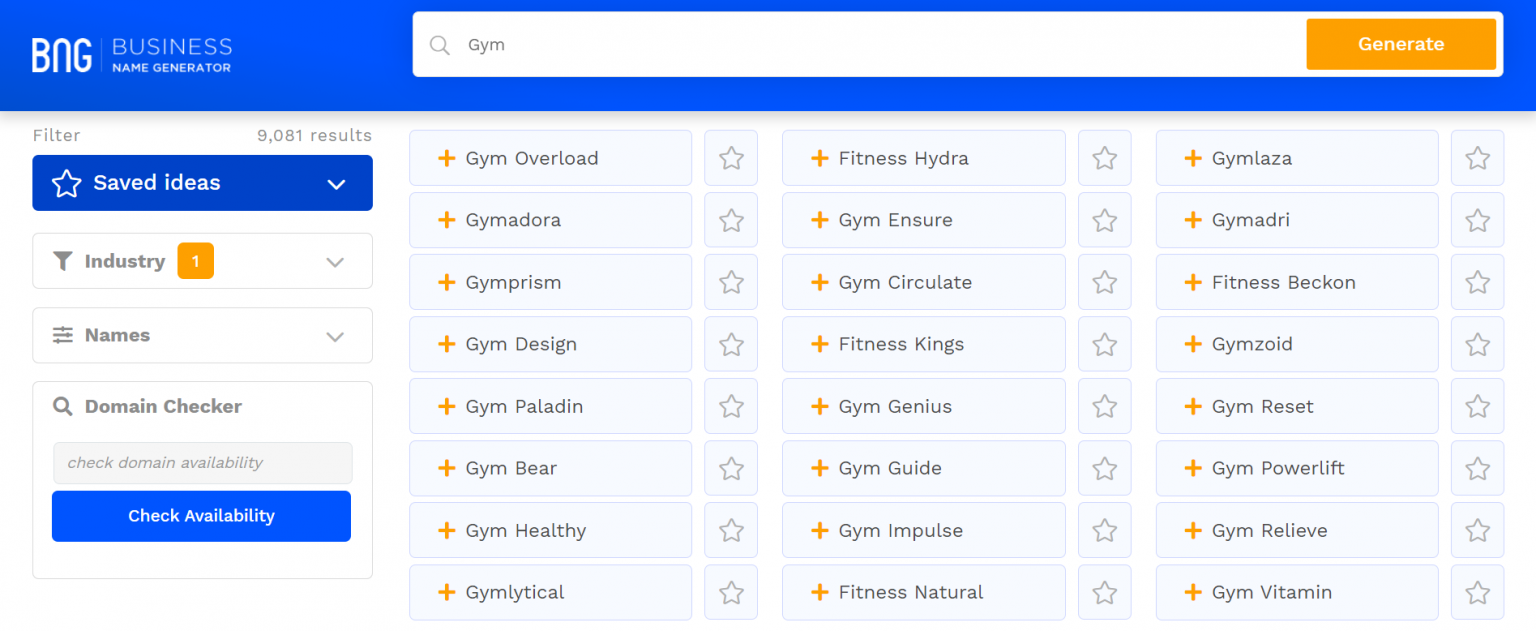A screenshot of the Business Name Generator (BNG) website, featuring a streamlined, modern design. The header displays a medium-dark blue gradient with the BNG logo in white on the left. Below the header sits an interactive text form pre-filled with the word "Gym" (G-Y-M) and an adjacent orange button labeled "Generate" in white text. The main content area has a clean white background with a color scheme predominantly consisting of white, blue, and medium gray. 

To the left, there's a navigation menu with sections like Saved Ideas, Industry, Names, Domain Checker, accompanied by a text box for checking availability, highlighted by a blue button labeled "Check Availability" in white text. 

On the right, a table showcases an array of AI-generated name suggestions in a three-column format. Visible within the screenshot are eight rows of name ideas, including "Gym Overload," "Fitness Hydra," "Gym Mazia," "Gym Dora," and "Gym Insure." Impressively, the generator has produced 9,081 results for the term "Gym."